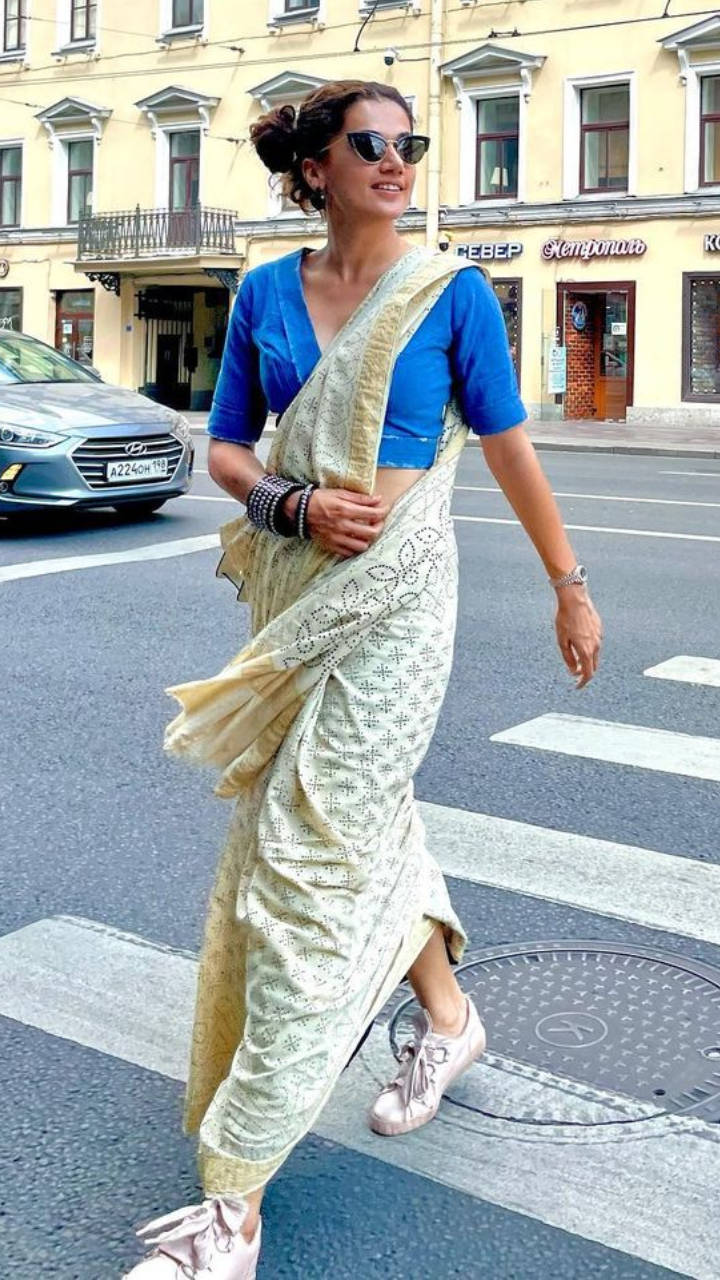This image captures a woman confidently striding across a pedestrian crossing on a road. She is attired in a cropped blue top with three-quarter length sleeves, complemented by black sunglasses and a collection of bracelets and a watch on her wrist. Her brown hair is neatly tied up at the back. She is wearing a distinctive white, ankle-length garment resembling a sarong or toga, and completes her outfit with white sneaker shoes. Notably, she is not wearing any socks. The woman glances towards the right side of the image as she walks. The road itself features white lines indicative of the crosswalk, with a manhole cover visible on the ground. In the background, a yellow building with numerous windows stands adjacent to the sidewalk. Additionally, a grey car waits on the left side of the image, its license plate partially visible.